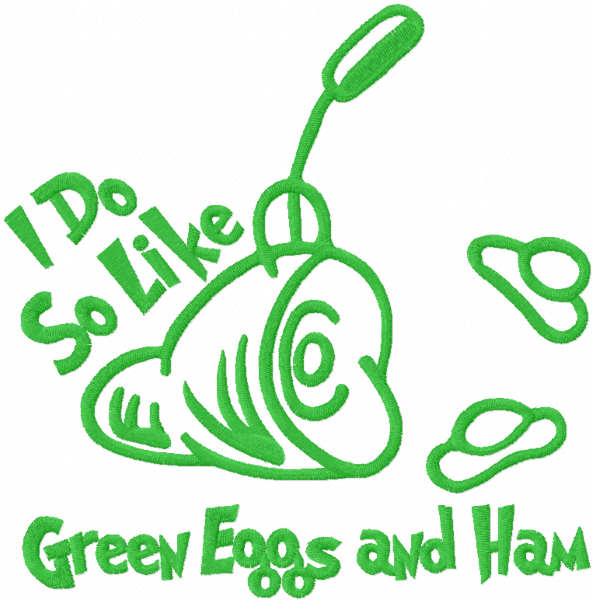This is a square, green-and-white graphic inspired by Dr. Seuss's style, featuring a bright green text and line drawings over a white background. At the upper left corner, it reads "I do so like" in a distinctive textured green font, reminiscent of a fibrous, patch-like texture. In the center, there's a simple, cartoon-like illustration of a ham with its front part sliced off and what appears to be a fork sticking into it. To the right of the ham, two green-drawn sunny side up eggs float in space. Below the central illustration, the phrase "green eggs and ham" is prominently displayed in the same green font.